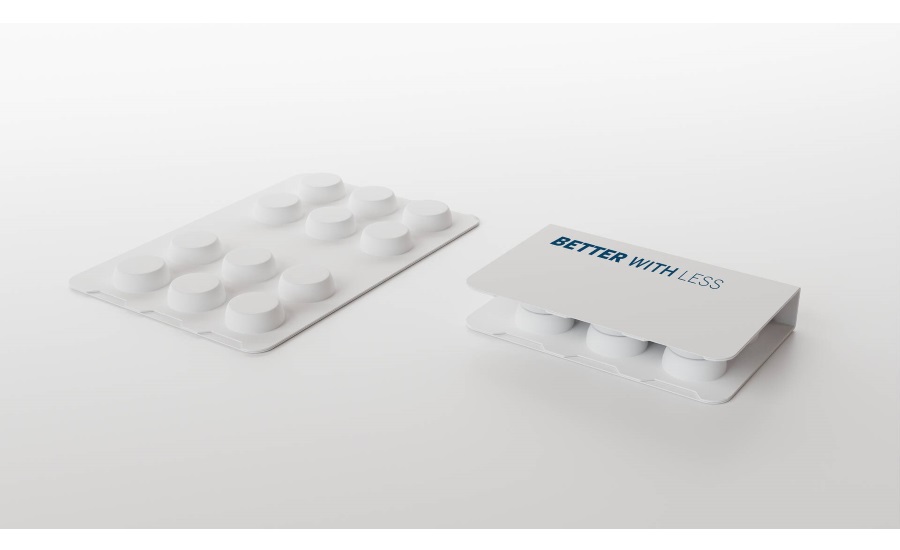In this detailed advertising photograph, the background is a clean white-gray. Two blister packs of pills are prominently featured, positioned diagonally toward the top right of the image. The left blister pack is laid flat, showcasing four columns and three rows of circular pill indentations, totaling twelve pills grouped into two clusters of six. The pack is white, with raised bumps indicating the pill housing.

On the right side, the same type of blister pack is displayed but folded in half. The inside portions, designed to hold the tablets, face inward, creating the appearance of two connected sections likely joined by a perforation. The outer, flat white container of this folded pack prominently features blue capital letters stating: "BETTER WITH LESS." The minimalistic design lacks any logos or ingredients lists, emphasizing the clean and straightforward nature of the product against the simple white backdrop.